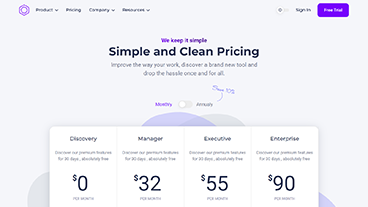This cropped screenshot showcases the pricing page for a productivity software. In the top left corner, there is a logo resembling a purple octagon, devoid of any textual name. Adjacent to this logo, there are four navigation categories labeled: Product, Pricing, Company, and Resources. On the far right, the page features a "Sign In" button alongside a prominently placed "Free Trial" button, highlighted in purple.

Centrally positioned at the top of the page is a headline in a small purple font that reads, "We keep it simple," followed by a bold declaration, "Simple and clean pricing." Directly beneath this is a smaller tagline in purple reading, "Improve the way you work, discover a brand new tool, and drop the hassle once and for all."

The pricing options are presented just below these descriptions, with a toggle button allowing users to switch between "Monthly" and "Annually"—the toggle in this screenshot is set to "Monthly." At the bottom of the screenshot, four pricing packages are displayed, categorized as Discovery, Manager, Executive, and Enterprise, each with the corresponding monthly prices clearly listed beneath them.